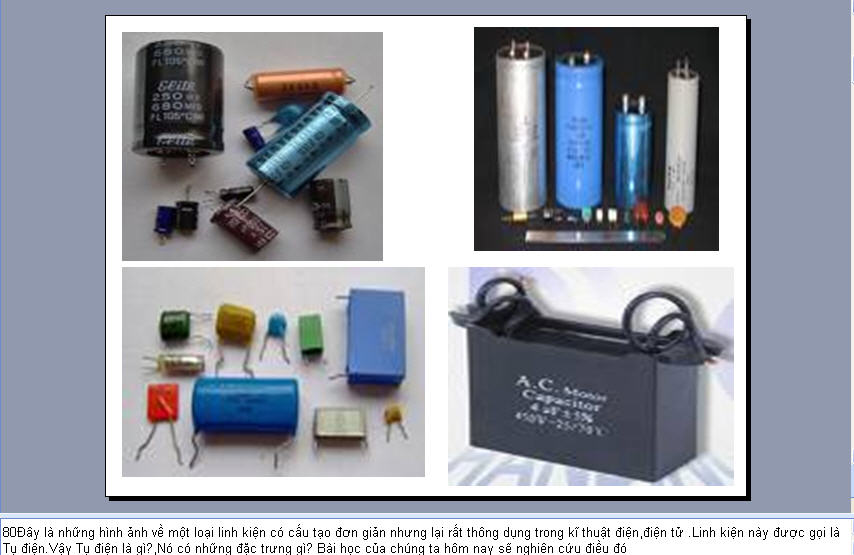The image consists of four separate photographs of electronic components, predominantly capacitors, arranged against a white background with a gray border. Each photograph showcases different types of capacitors and related electronic items. 

In the upper left-hand corner, there are multiple capacitors, including one large black capacitor and a smaller blue one, among others, lying scattered. These capacitors vary in size and voltage, with visible wires extending from them. The upper right-hand corner features another set of capacitors, neatly standing upright in a vertical position, including silver, blue, and gray ones. 

The bottom left-hand corner displays about half a dozen smaller capacitors of various shapes, such as cylindrical and rectangular, neatly laid out against a gray-white background. On the bottom right-hand corner, there is a gray metal box, with white text reading "capacitor" on it, presumably for storing some of the components. 

Below the entire image, there is text written in Vietnamese. The image as a whole provides a detailed look at an assortment of electronic components, highlighting the diversity in types and arrangements of capacitors.